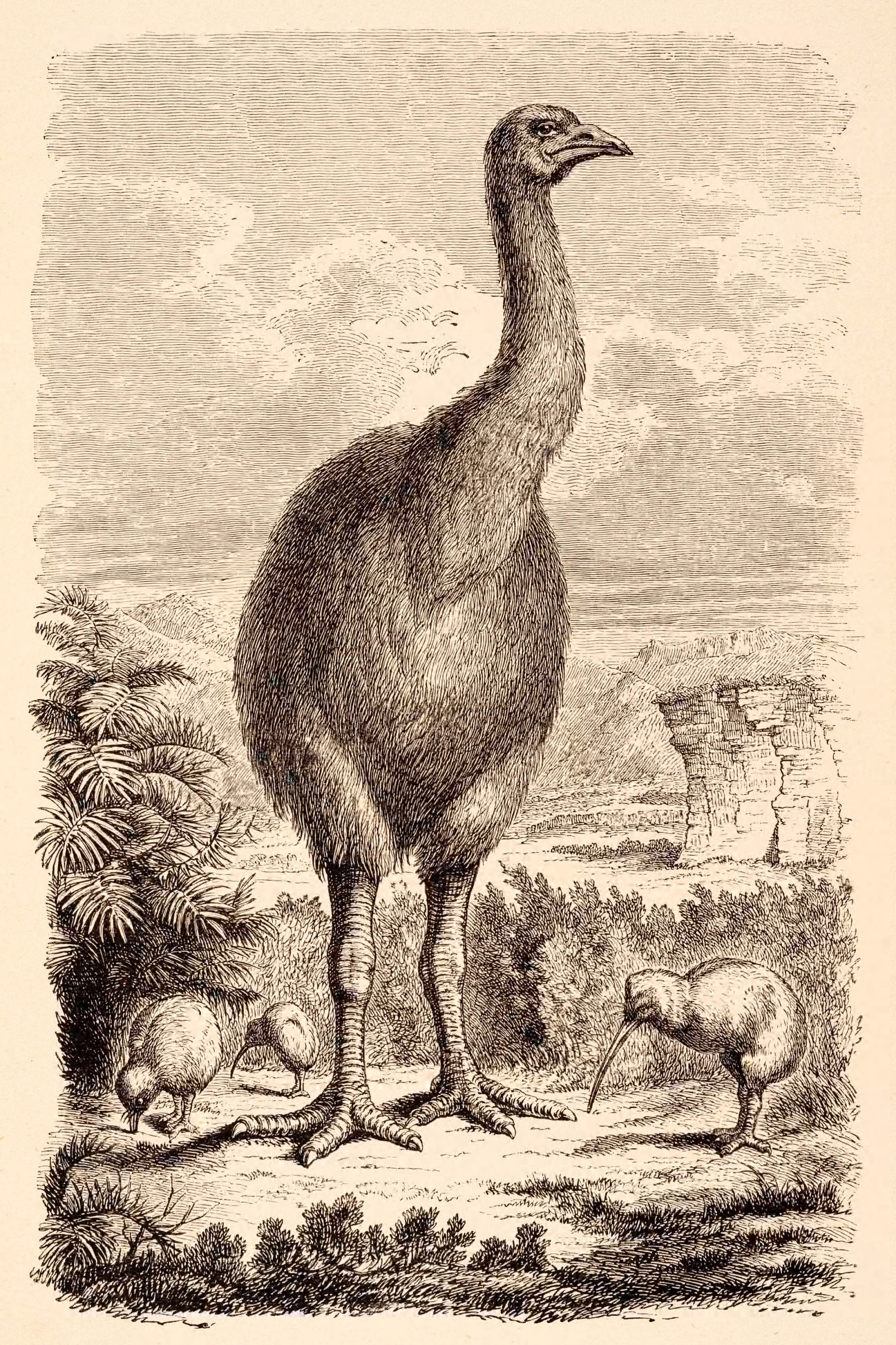The artwork is a detailed black and white ink drawing on tan paper, depicting a scene dominated by a large, ancient bird that could be a kiwi or a similar species. This prominent bird, with its long neck and imposing stature, stands at the center of the composition, overshadowing several smaller birds below it. These smaller birds, which have long beaks and are engaged in pecking at the ground, contribute to the dynamic interaction within the scene. The environment around them is rich with dirt, grass, and lush tropical-style bushes, setting a naturalistic background. In the distance, a rocky cliff and mountain range add depth to the illustration, suggesting a vast and varied landscape. The drawing captures a moment of stillness amidst nature, highlighting the protective stance of the large bird possibly overseeing the smaller ones. The monochromatic palette and intricate line work emphasize the textures and forms of both the birds and their surroundings.